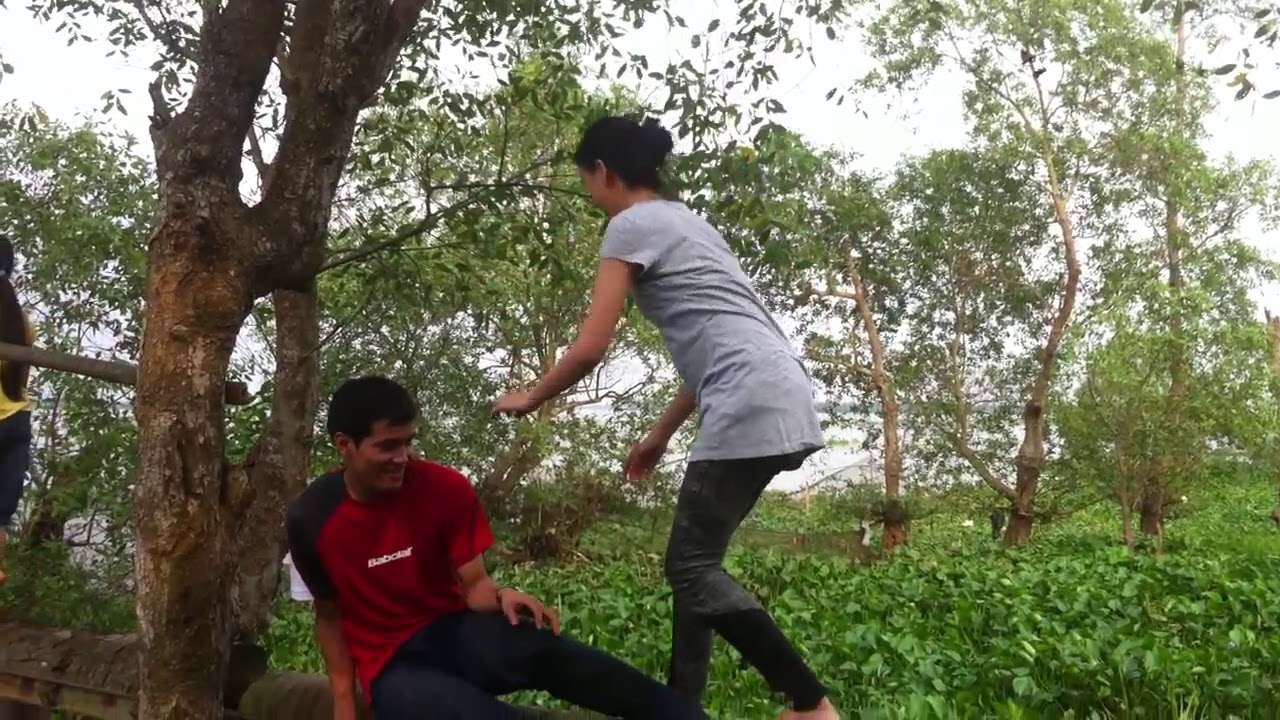In this horizontal photograph, two main subjects engage in a dynamic scene set in a lush, wooded area. At the base of a multi-trunk tree on the left, a man with dark hair and tan skin sits, clad in a red shirt and black pants. In the center, a woman with dark hair, wearing a gray shirt and gray leggings, reaches out towards the seated man. Her posture suggests an interaction, perhaps a game or playful moment. The backdrop showcases a dense array of trees with small trunks and abundant green leaves. Patches of gray sky peek through the canopy, indicating overcast weather. A hint of another person is visible at the far left edge of the image but is incomplete. The ground is covered in green foliage, contributing to the overall verdant ambiance.